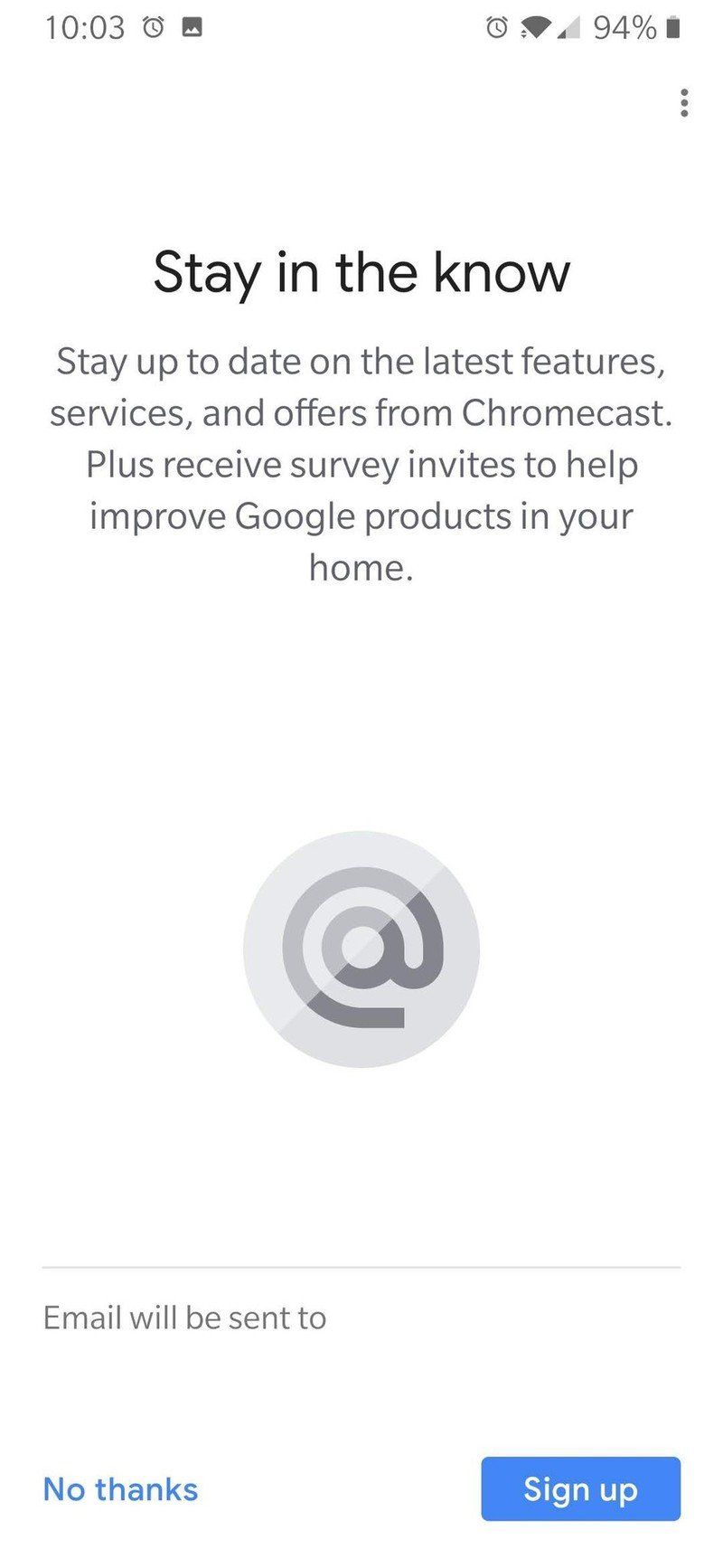This screenshot captures a cell phone interface at the top displaying the current time, signal strength, Wi-Fi connectivity status, battery level, and a three-dot menu icon. The background of the image is predominantly white with black text.

At the center, a prominent title reads "Stay in the know." Below the title, a message board encourages the user to "Stay up to date on the latest features, services, and offers from Chromecast. Plus, receive survey invites to help improve your Google products in your home."

Further down, an app icon is depicted within a gray circle. A horizontal divider follows, leading to a section that indicates an email will be sent to a specific address. At the bottom of the screen, two buttons provide the user with options: "No thanks" and "Sign up." The "Sign up" button is currently highlighted, while the "No thanks" button remains unselected.

Overall, this image details a cell phone screenshot displaying a sign-up prompt for updates and survey invitations related to Chromecast features and offers.